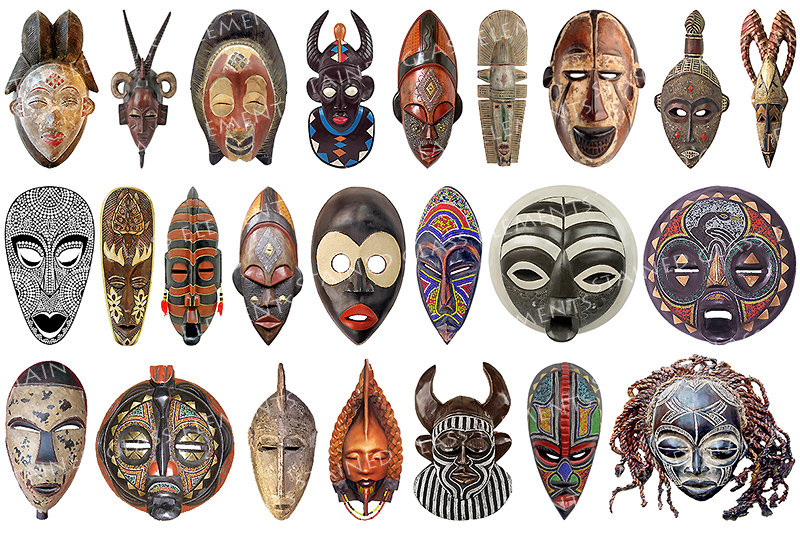This photograph showcases approximately 25 traditional, indigenous-looking mask plaques or sculptures, meticulously arranged in three rows. Each row contains an array of unique masks, varying in shape and design but predominantly oval or round. Crafted from materials like stone or wood, these masks are intricately decorated with vibrant, earthy tones along with reds, blues, greens, blacks, and whites. The masks exhibit a spectrum of expressions, with differing states of eyes, indicating varied emotions from being awake to asleep.

The first row begins with a series of masks featuring a mix of brown, red, and white hues. Including a red and tannish-colored mask and a striking brown, blue, and white mask. Some masks in this row have slender, pointed chins and vivid geometric patterns that lend them an almost alien appearance. More masks display dark brown paired with lighter shades like white or tan.

In the subsequent rows, the diversity in color becomes more evident with combinations of red and orange, green and orange, and black and white. Some masks are simpler with solid hues, while others boast a complex interplay of numerous colors. Noteworthy are the multicolored masks, one with bronzed elements juxtaposed with black, and another black and white-striped mask adorned with horns. One particularly fascinating mask features yarn for hair, combining black, white, and brown shades.

Overall, the collection exudes a rich cultural heritage, with each mask embodying unique artistic expressions through its color palette, decor, and form.